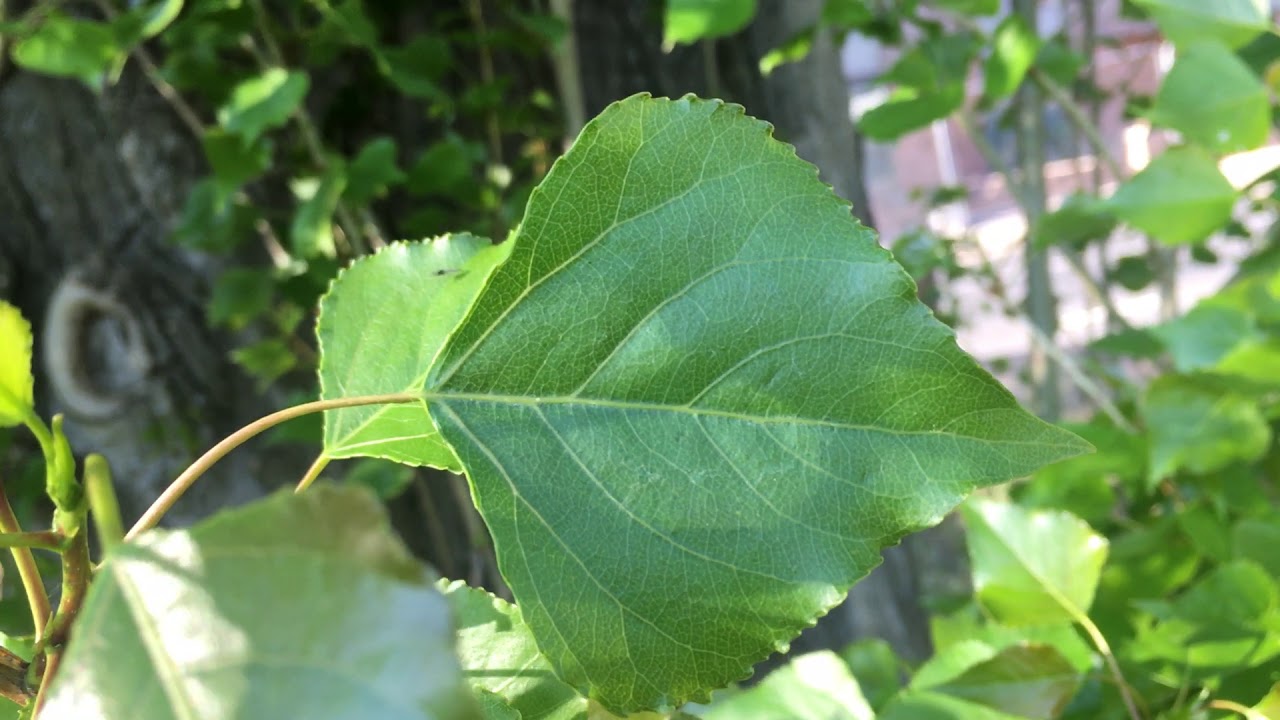This landscape photograph features a vivid green leaf, prominently positioned in the center as the main focus. The leaf, lying on its side, is somewhat diamond-shaped with serrated edges that come to a pointed tip aiming towards the right side of the image. The stem of the leaf extends from the center towards the bottom left corner, adding to the dynamic composition of the scene. The background, beautifully blurred to emphasize depth, consists of layered leafy vegetation and a dark gray tree trunk with a large knot on the left side. Additionally, shadow patterns play across the leaves, illuminated by sunlight filtering through the canopy. Far in the background, just faintly, there appears to be an apartment building in the upper right-hand corner, suggesting the setting is a wooded area in daylight, filled with nature’s vibrant hues and textures.